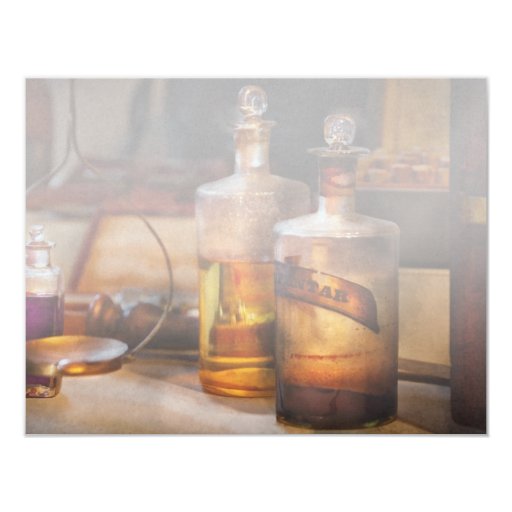This image showcases a vintage-styled scene with two large glass bottles prominently placed on a light brown wooden counter. These bottles are fitted with glass stoppers. The bottle on the right contains a brown liquid and bears a brown label partially reading "N-T-A-R." The bottle on the left is partially filled with a yellowish liquid and lacks any label. The overall image is enveloped in a smoky, hazy ambiance, giving it an antiquated, almost faded aesthetic, reminiscent of an old photograph. To the left of the large bottles, a smaller glass bottle—also with a glass stopper—holds a purple liquid, filling it about three-quarters full. Additionally, in the bottom left corner, there is a round metal utensil, and behind the bottles, a wooden tool or frame is partially visible among the other indistinct items. The color palette of the scene includes varying shades of brown, white, clear, and hints of purple and yellow, suggesting a cellar-like or rustic home setting.